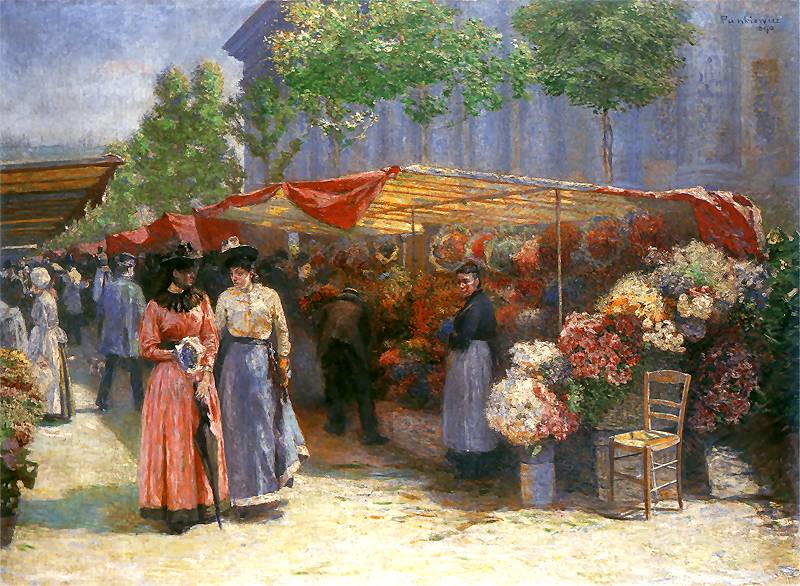This detailed oil painting captures a bustling outdoor market scene reminiscent of Victorian times. On the right side, a vibrant flower stall covered with a red cloth is laden with an array of colorful flowers, including white, red, orange, purple, and blue blooms. Beneath the stall, a woman in a blue dress stands beside an empty chair, gazing at two other women strolling by. One of these women wears a blue dress with a white top and a black hat, while the other is dressed in red, holding an umbrella and possibly some flowers. Both women don Victorian-style hats, contributing to the historical ambiance, with their long skirts and blouses reflecting the fashion of the era. In the background, numerous people traverse the market, enjoying their day amidst the rows of stalls that extend into the distance. The upper part of the painting features lush green trees that stretch across the scene, with a glimpse of blue sky peeking through. The ground, possibly dirt or cobblestone, stretches out beneath the bustling market, adding to the rustic charm. A signature is visible in the top right corner, affirming the artist's handiwork.